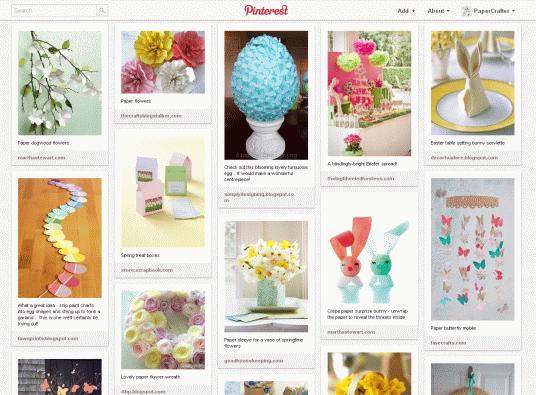This image captures a Pinterest webpage, displayed in a horizontal rectangular format. The iconic Pinterest logo is prominently featured at the top in red font against a white background, which forms a horizontal white rectangular section distinct from the rest of the image.

Below the header, the page showcases a variety of images, organized into several vertical rectangular sections. These images are visually engaging and appear to focus on a springtime or Easter theme, predominantly featuring flowers and bunnies. 

1. The first image in the sequence displays a light green background, adorned with hanging flowers. Beneath the image, there is some text, along with potentially clickable links leading to websites for further exploration.

2. The second image features a quartet of flowers, arranged against a similarly verdant backdrop.

3. Moving across the top row, the next image showcases a creative arrangement that resembles an egg made from blue flowers, all nestled within a white vase.

4. Adjacent to this is an image depicting an elegant table setting, festooned in hues of pink and green, complete with decorative flowers.

5. Following this is an image encased in a yellow border, featuring a piece of china with a white interior. Centered on the plate is a napkin folded into the shape of bunny ears, complemented by a background of yellow flowers, enhancing the festive feel.

Further down the page, more images continue the spring and bunny theme. Notably, there is a charming image of two bunnies, one with a red head and the other with a green head, both sporting floppy ears.

Each of these images is clickable, providing various inspirations and ideas that capture the essence of springtime celebrations.